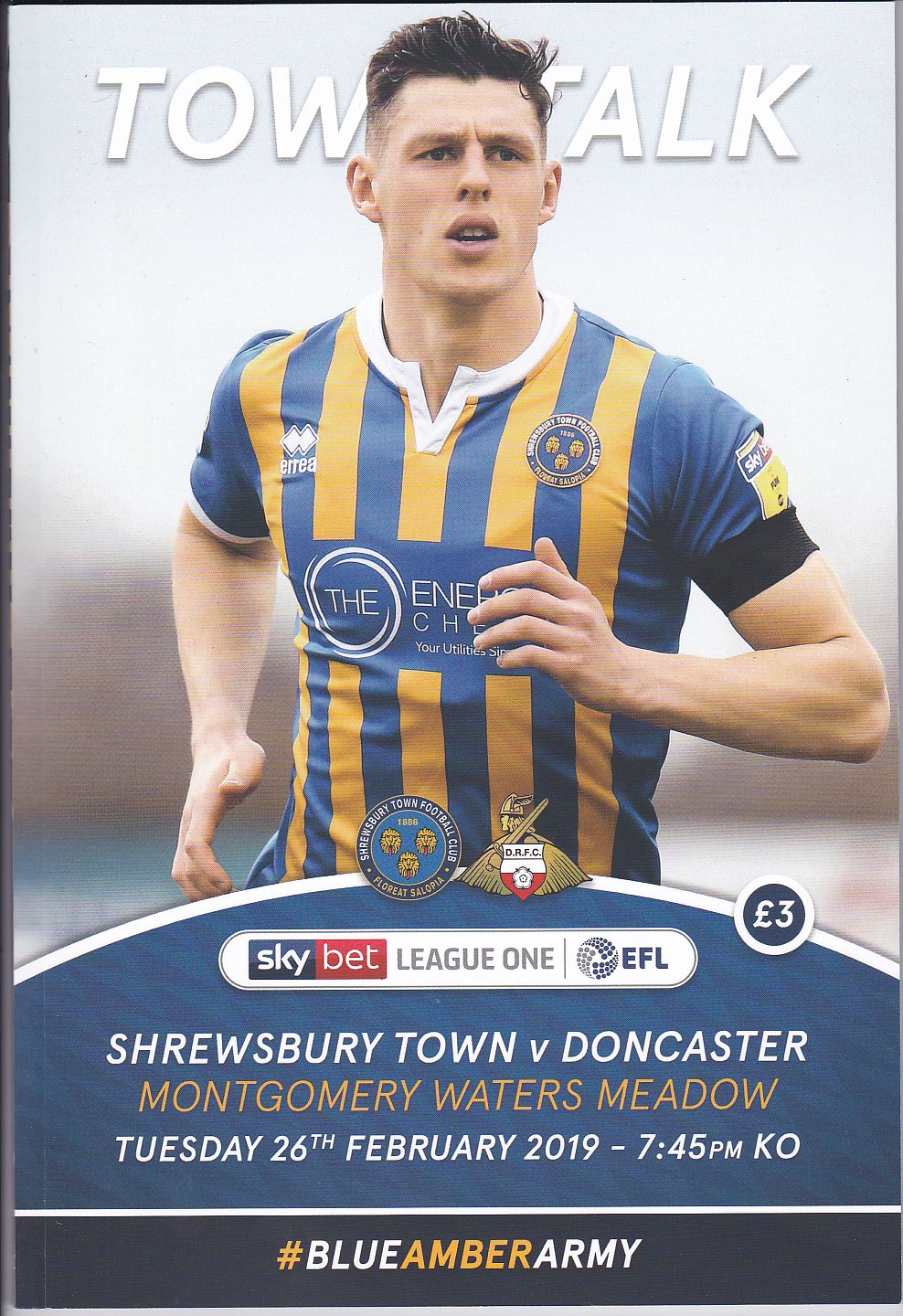The vertical rectangular advertisement poster promotes a soccer game, featuring a central image of a young, dark brown-haired player in a blue and yellow striped jersey, captured mid-run. The top half of the uniform displays a couple of badges, though part of the central text on the jersey is obscured by the player's hands. Above the player's head, large white letters spell "Town Talk," though the athlete’s head blocks some of the text, making it partially hidden. Below the player, a blue area includes emblems and the detailed match information: "Shrewsbury Town vs Doncaster, Montgomery Waters Meadow, Tuesday 26th February 2019, 7:45 pm." A horizontal black strip at the bottom features the hashtag "#BlueAmberArmy."